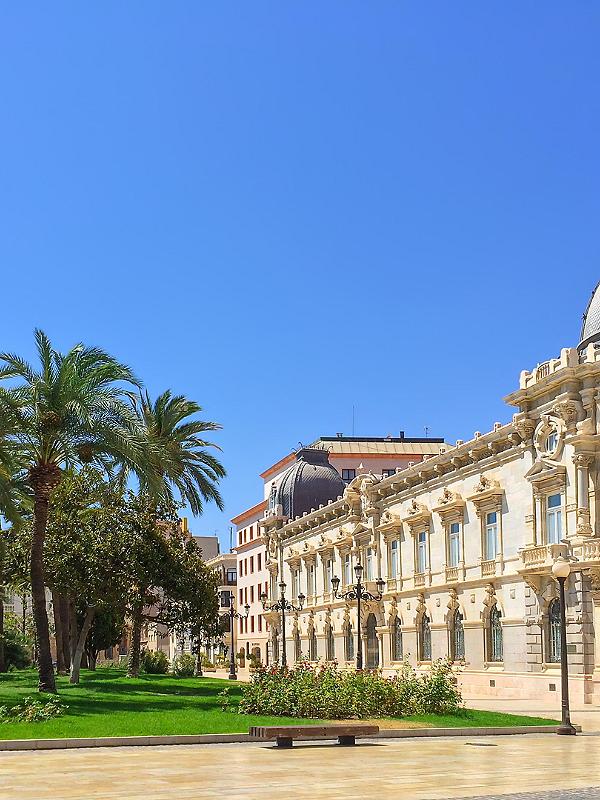The photograph captures a serene outdoor scene centered around an old, ornate two-story building that resembles a palace, possibly located in a tropical or subtropical region such as Florida or a European country. The sky above is a vibrant shade of either powder blue or deep ocean blue, with no clouds in sight, indicating a bright, clear day. In the foreground lies a meticulously maintained patch of deep green grass, bordered by neatly arranged lampposts and shrubberies.

Palm trees tower above the building, adding to the tropical ambiance, and they are positioned predominantly on the left side of the image. A small, wooden bench sits centrally within a tiled, mosaic-like plaza or town square. This bench is framed by a well-manicured area with concrete step-over bricks and lush plants, contributing to the overall orderly and picturesque environment. Behind the palace, a few more modern three- to four-story buildings are visible, complementing the historical structure with their contrasting architectural style. The palace itself features beige-white stones, ornate columns, and a couple of bluish domed roofs, adding to its grandeur and historic charm. Notably, there are no people present in the photograph, allowing the viewer to fully appreciate the tranquil and well-maintained setting.